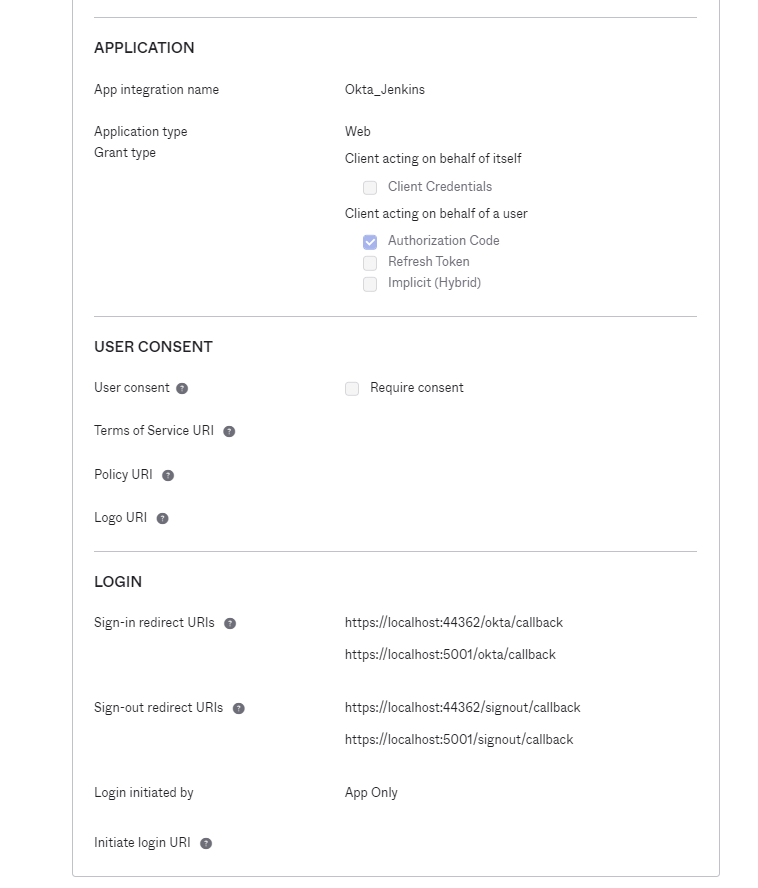Here is a meticulously detailed caption for the described image:

---

The image features a detailed, organized sheet bordered by a thin gray line that encompasses the perimeter. The interior of the sheet is divided by several horizontal lines which segment the content into distinct informational categories. At the top, bold black text prominently reads "Application." Below this, the sheet details various integration specifics, starting with "App Integration Name: Okta_Jenkins," followed by "Application Type: Web."

Further down, the sheet lists authorization methods with a specified grant type of "Client acting on behalf of itself: Client Credentials" and other options including "Client acting on behalf of a user: Authorization Code" — marked with a check — as well as "Refresh Token" and "Implicit (Hybrid)."

The next section focuses on user-based information labeled "User Consent." This part includes fields for "Terms and Services URI," "Policy URI," "Logo URI," and an option for "Require Consent" accompanied by a checkbox.

Additional details encompass login specifics, such as "Login/Sign-In Redirect URIs," "Sign-Out Redirect URIs," and a question regarding login initiation labeled "Login initiated by Initiation Login URI?" There are several localhost callback URLs listed below this query, tailored for various setup requirements.

At the bottom of the sheet, the term "App Only" is clearly displayed, finalizing the detailed capture of integration and user management information.

---